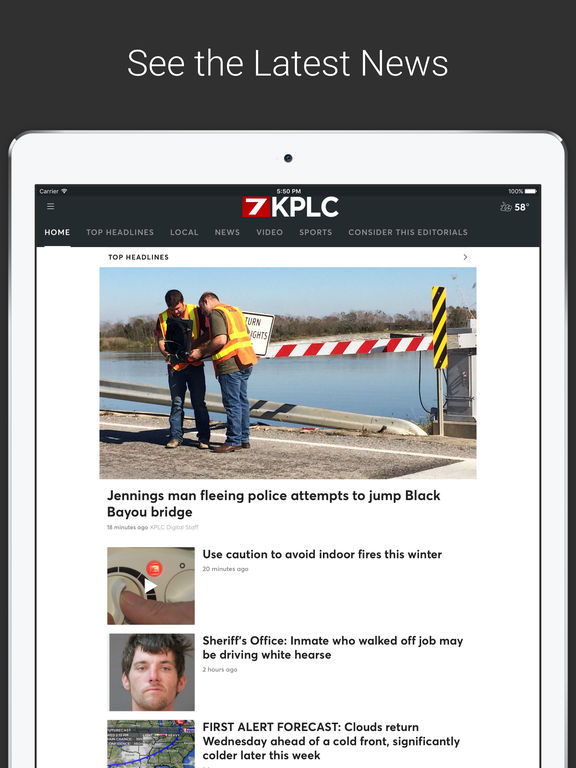The image features a sleek white tablet placed against a stark black background, showcasing a news application screen. The screen reads "Latest News" in bold white text at the top. On the left corner of the tablet's screen, icons indicate a Wi-Fi connection with three full signal bars and a status of "Carrier." In the center, the device displays the current time as 5:50 p.m., accompanied by a battery indicator showing full charge at 100%, and the local temperature of 58°F.

At the top of the screen, a black header bar lists several navigation options: "Home," "Top Headlines," "Local News," "Video," "Sports," "Editorials," and others. Below this bar, the section titled "Top Headlines" begins with a news photo featuring two men wearing high-visibility construction vests.

The headlines displayed are as follows:

1. "Jennings man flees police, attempts to jump Black Bayou Bridge" by Joe Yo.
2. "Use caution to avoid indoor fires this winter."
3. "Sheriff's Office: Inmate who walked off job may be driving white hearse."
4. "First Alert Forecast: Clouds return Wednesday ahead of cold front, significantly colder later this week."

The overall tone of the image is modern and crisp, highlighting the tablet as a portal to the latest local and national news updates.